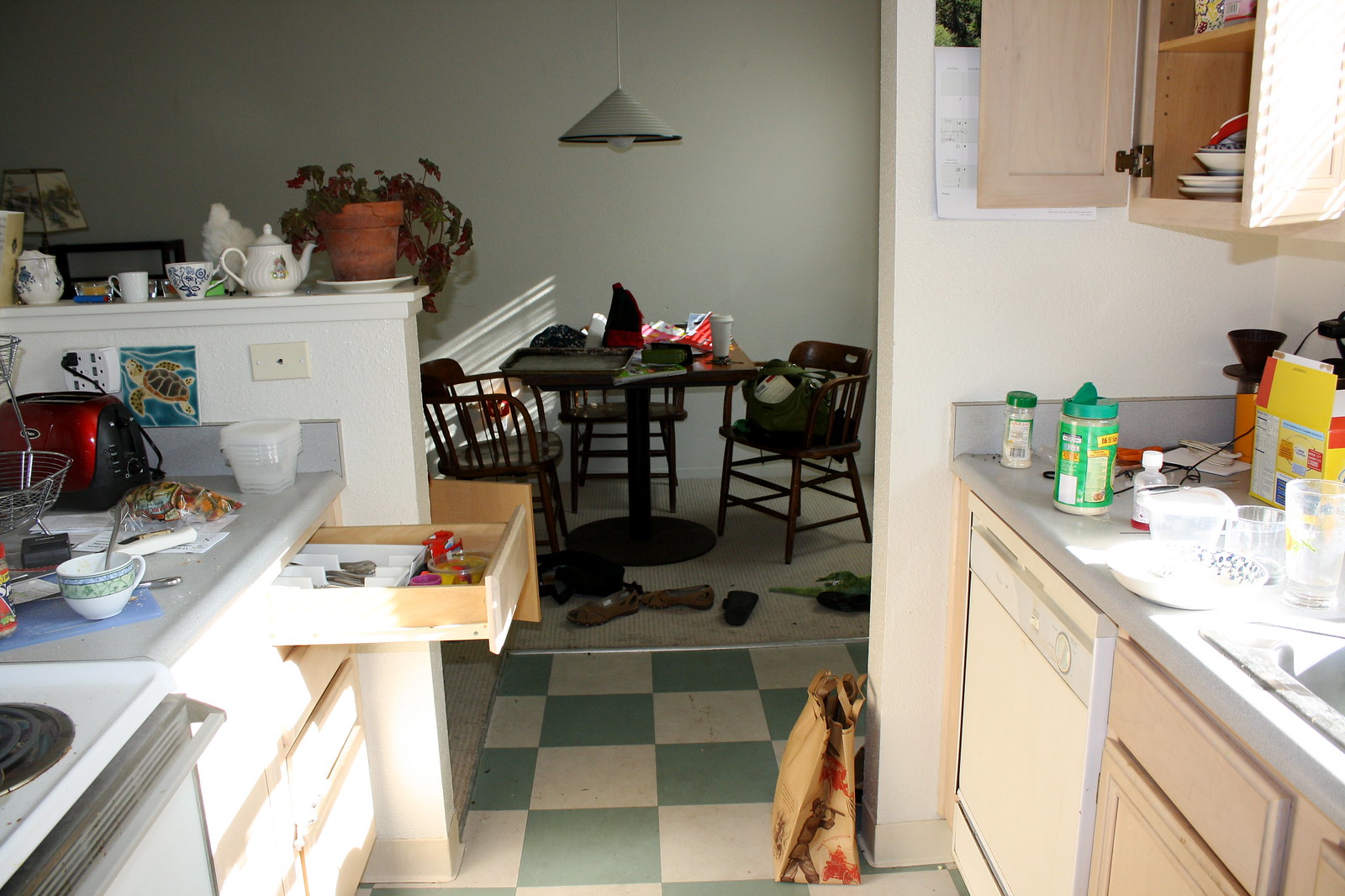The photo captures an interior view from a messy kitchen into an adjoining dining room. On the left side of the image, the kitchen features a piece of electric stove protruding into the frame, identifiable by its white top and black coils. The gray, plastic laminate countertop is cluttered, holding various items including a wire basket, a red toaster plugged into the wall, and a stack of square plastic storage containers. The countertop continues above a white dishwasher with a conspicuous turn dial.

A drawer in the kitchen has been left ajar, revealing a plastic silverware holder with scattered utensils, surrounded by miscellaneous knickknacks. The wall displays a picture of a sea turtle, painted in shades of brown and green, adding a touch of marine life to the space.

The checkered kitchen floor consists of alternating squares in bluish-gray and white. Positioned on the floor is a brown Trader Joe's grocery bag, illustrated with a male cartoon character looking through a scope and adorned with red leaves. The overall scene suggests a well-used, albeit chaotic, kitchen environment bridging into a presumably more orderly dining area.